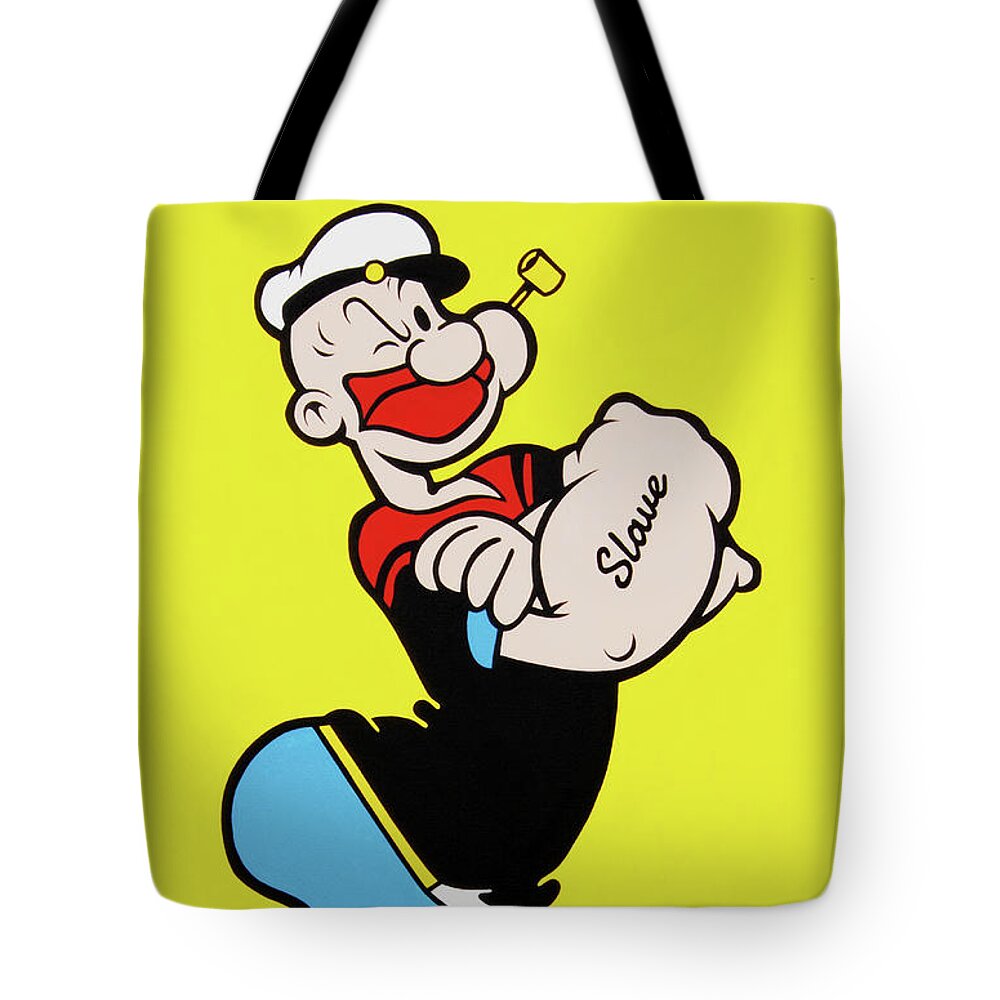The image features a bright neon yellow tote bag set against a pure white background, with black straps extending upward from either side of the bag. The front of the bag prominently displays a CGI-rendered cartoon character strikingly similar to Popeye. He is wearing a black shirt with a red design across the shoulders, blue pants, and a white sailor's cap with a black brim. Popeye's posture is notably arched backward, with his large forearms crossed in front of his chest. One forearm bears the word "SLAVE" in black text. His facial features include a large round nose, red lips, and a yellow pipe protruding from his mouth. He is winking, with a curly black eyebrow accentuating his expression. Overall, the bag's vibrant color and detailed character depiction make it eye-catching and memorable.